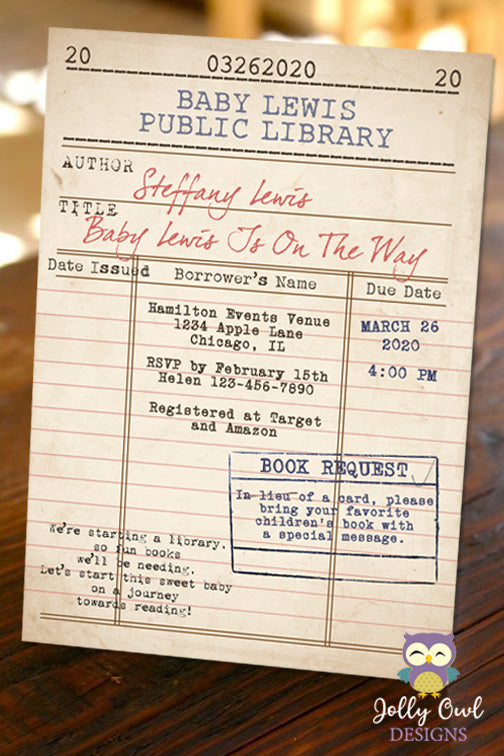The photograph showcases a library checkout card placed on a rustic wooden table, slightly tilted to the left. The card, printed on white paper, features a black outlined section at the top where the numbers "20," "03262020," and "20" are displayed. Below this, "Baby Lewis Public Library" is written in blue lettering, followed by hand-written red text naming the author as "Stephanie Lewis." Further down, the title "Baby Lewis is on the way" is also hand-written in red. The structure of the card includes columns labeled "Date Issued," "Borrower's Name," and "Due Date," with the borrower's name listed as "Hamilton Events Venue, 123 Apple Lane, Chicago, Illinois." An RSVP is requested by February 25th, and the location is registered at Target and Amazon. The due date is stamped as March 26, 2020, at 4 p.m. A blue rectangle at the bottom right reads "Book Request," urging guests to bring a favorite children's book with a special message instead of a card. Additionally, there is a small logo at the bottom featuring a cartoon owl and the text "Jolly Owl Designs."